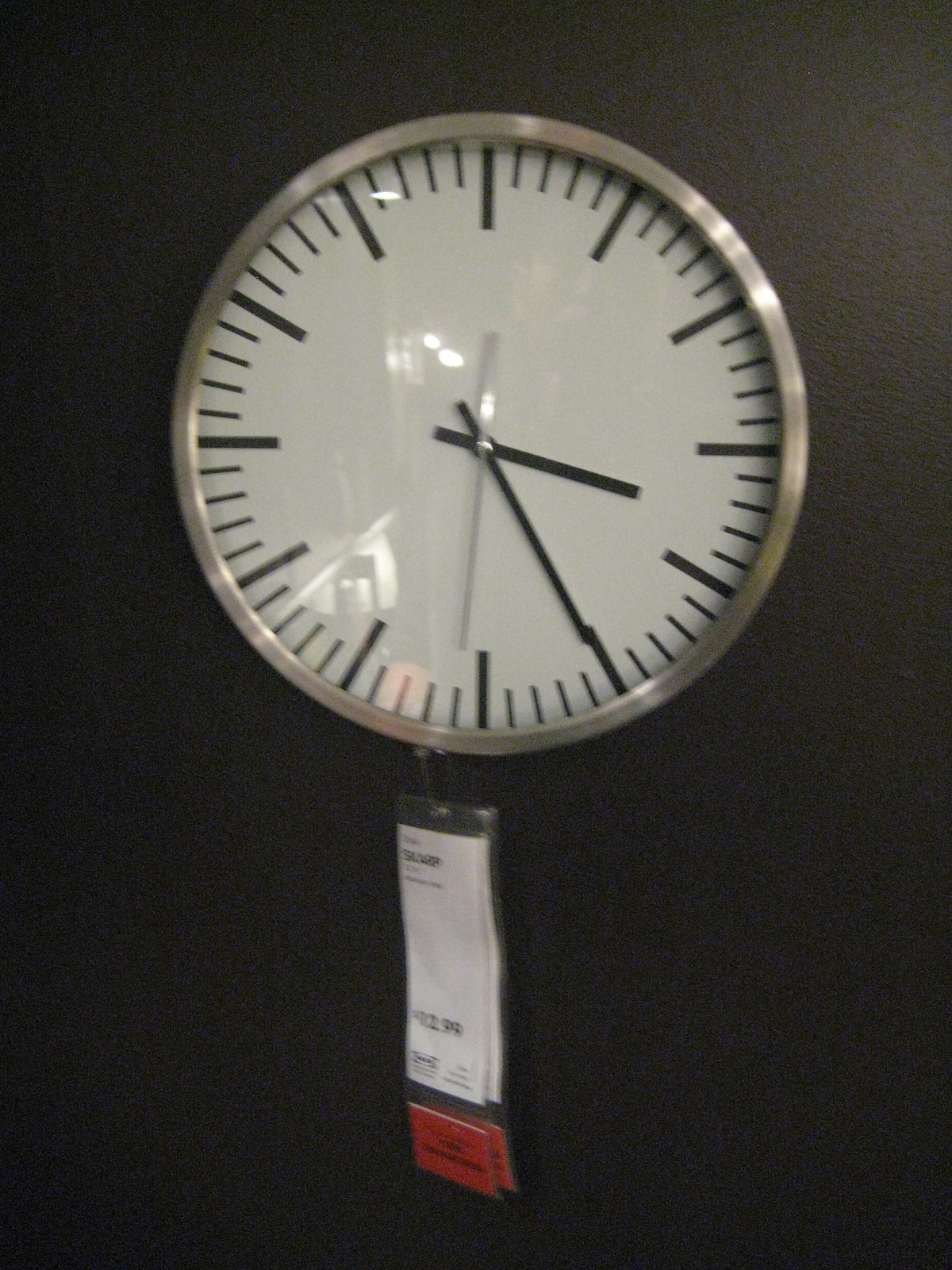This image showcases a minimalist wall clock prominently displayed on a retail display wall. The clock features a sleek steel case encircling a clean white face. It is designed with simple black hour and minute hands, and a contrasting silver second hand, contributing to its modern aesthetic. Notably, the clock eschews traditional numerical markers, opting instead for longer lines to denote the hours and shorter lines for the minutes, enhancing its minimalist appeal. Below the clock, a tag hangs, likely indicating that this is a product available at Ikea, with a clearly visible price of $12.99. Additionally, a red tag beneath the product price likely provides information on the specific aisle where customers can find the clock within the store.